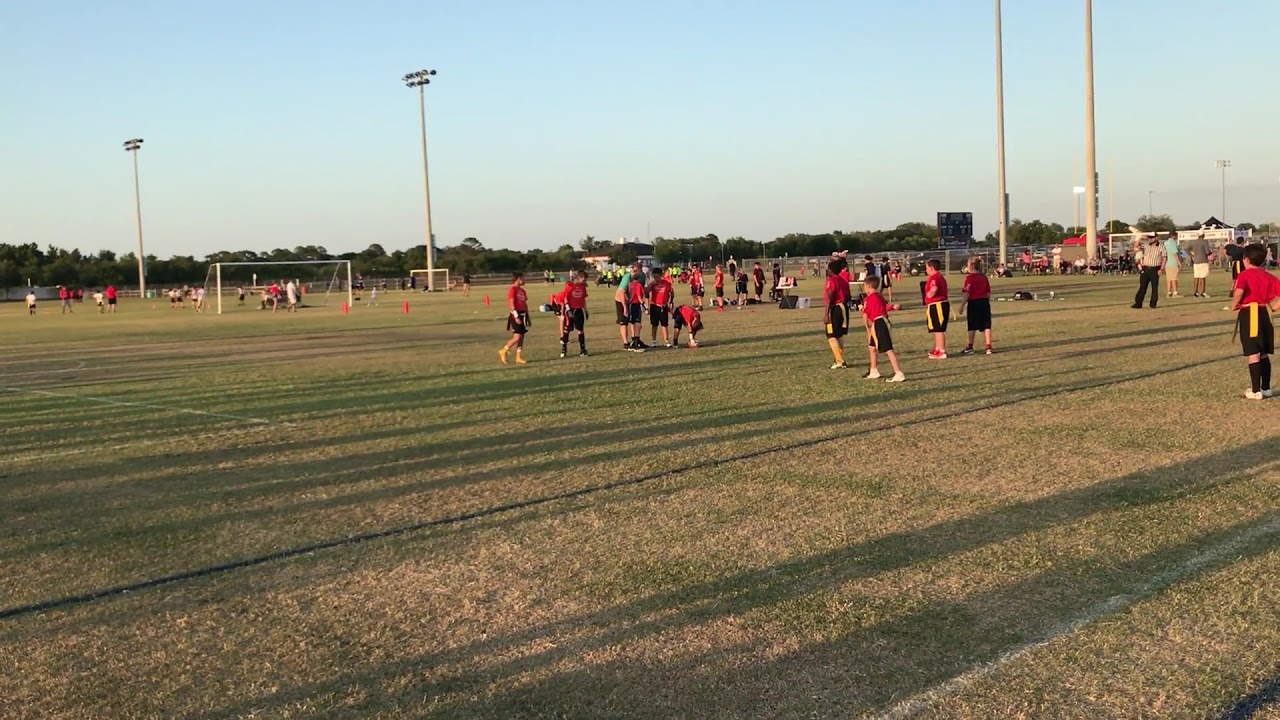This photograph, taken outdoors on a sunny day with elongated shadows suggesting it’s near dusk, captures a large open soccer field dotted with splotches of green and dry brown grass. A faint white painted stripe runs from the bottom towards the right-hand side of the image. Numerous child players wearing red short-sleeved shirts, black shorts, and yellow bands tied around their waists are scattered across the field, seemingly engaged in a soccer camp or possibly playing flag football, though no soccer balls are visible. In the background to the left, a soccer goal is discernible amidst clusters of people. A ridge of trees spans the midline from left to right, framed by tall stadium lights in the center. Above it all stretches a bright blue sky, enhancing the vibrant outdoor scene.